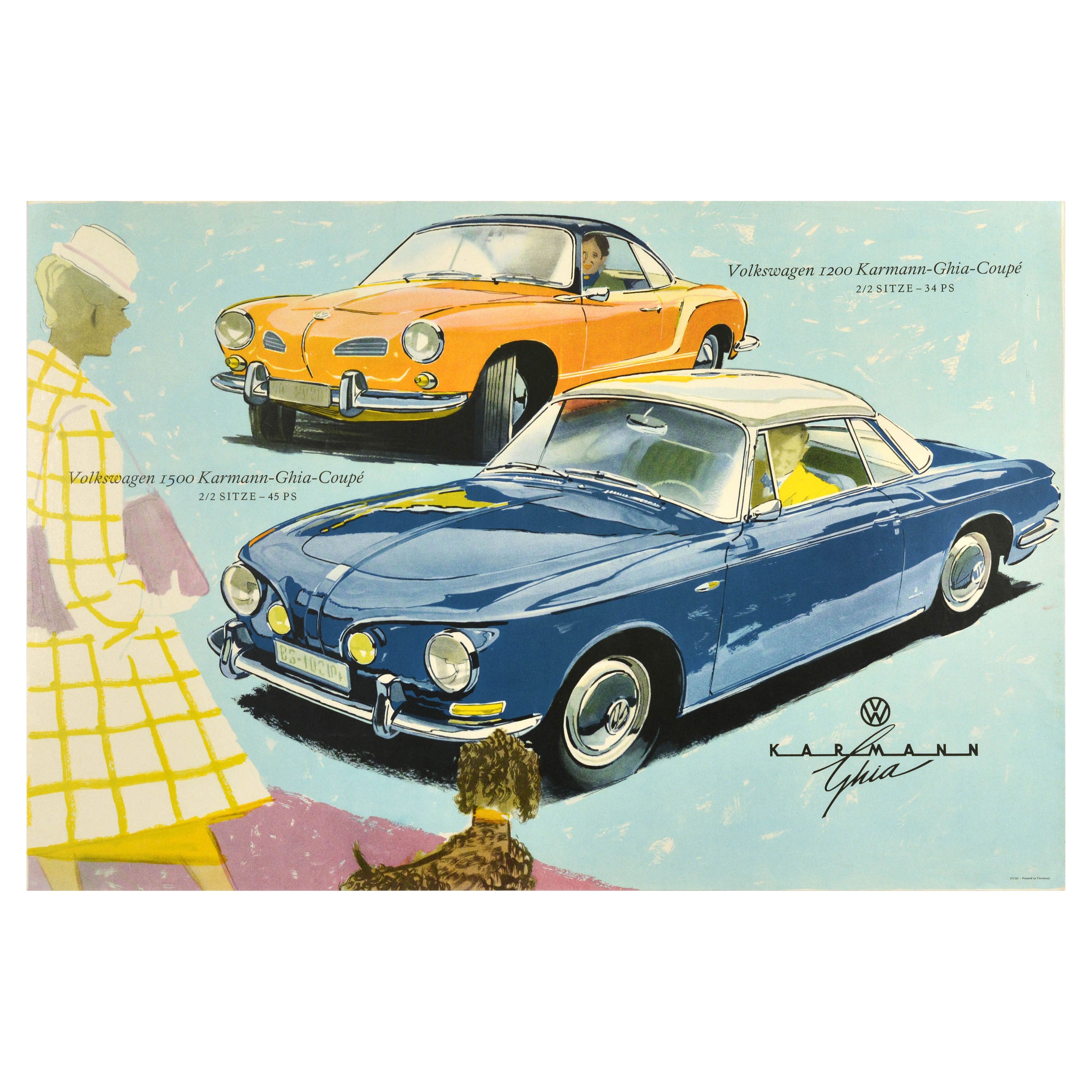This image is an animated, horizontal rectangular ad showcasing two vintage cars on a light blue background. The top middle features an orange, two-door Volkswagen 1200 Karmann Ghia Coupe, subtly facing left, with small black writing to its right that reads "Volkswagen 1200 Karmann Ghia Coupe" followed by "2 out of 2 seats, 34 PS." Below and slightly to the right, there's a larger, blue, and white-topped two-door Volkswagen 1500 Karmann Ghia Coupe, also facing left. Above the hood and to the left of this blue car, it says "Volkswagen 1500 Karmann Ghia Coupe" followed by "2 out of 2 seats, 45 PS." To the left of these cars stands a woman in a white coat with yellow lines, holding a purple purse over her right shoulder, and wearing a white hat, gazing at the cars. A brown dog with curly hair sits at her feet, facing the cars. At the bottom right corner, underneath the driver's door of the blue car, there's a Volkswagen symbol with "Karmann" written beneath it in black, and the word "Ghia" in italics below that, accompanied by an illegible signature.